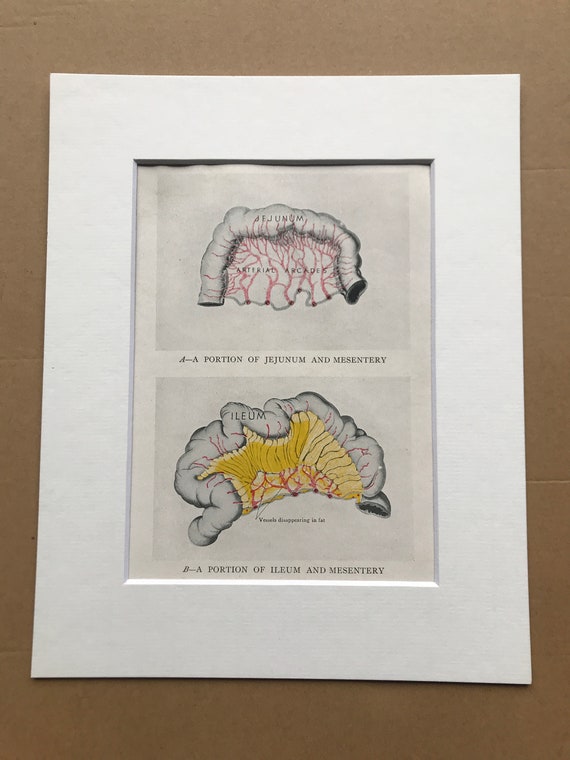This detailed photograph captures a page from a scientific book, specifically an anatomical illustration of parts of the human gastrointestinal system. The image is set against a brown backdrop, likely an unfolded piece of cardboard, with visible fold marks, adding a rustic touch. It is meticulously mounted within a thick white mat, framed by a brown border, ready for display.

The illustration is divided into two panels stacked vertically. The top panel, labeled "A," features a color drawing titled "Portion of Jejunum and Mesentery." It depicts a gray, arched segment of the jejunum, a part of the small intestine, accompanied by intricate red artery arcades branching prominently through the mesentery below.

Beneath it, the bottom panel labeled "B" is titled "Portion of Ileum and Mesentery." This illustration shows a similar gray section of the ileum, another part of the small intestine, surrounded by a yellow area within the mesentery. The yellow region is interwoven with both black and red veins, with a specific pointer indicating "vessels disappearing in fat." The entire matted illustration sits elegantly on a plain tan background, highlighting the detailed anatomical elements.